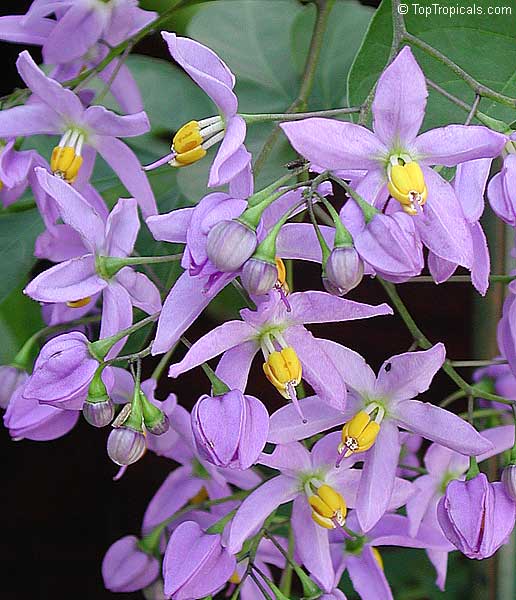In this photograph from toptropicals.com, vibrant lilac-purple flowers with five delicate petals and striking yellow centers burst forth in various stages of bloom. Some flowers are fully opened, proudly displaying their intricate structures, while others remain closed as buds, hinting at their eventual beauty. The flowers, likely growing from a tree or bush, emerge amidst a backdrop of dark stems and green leaves, suggesting a dense, lush environment. The natural light illuminates the scene gently, indicative of a slightly overcast day that softens the overall brightness. The meticulous detail of the yellow centers, which appear in five-part segments, further captivates the viewer's attention. The presence of a subtle watermark in the top right corner hints that this image may serve as a product display, possibly offering a glimpse into the horticultural treasures available on the website.